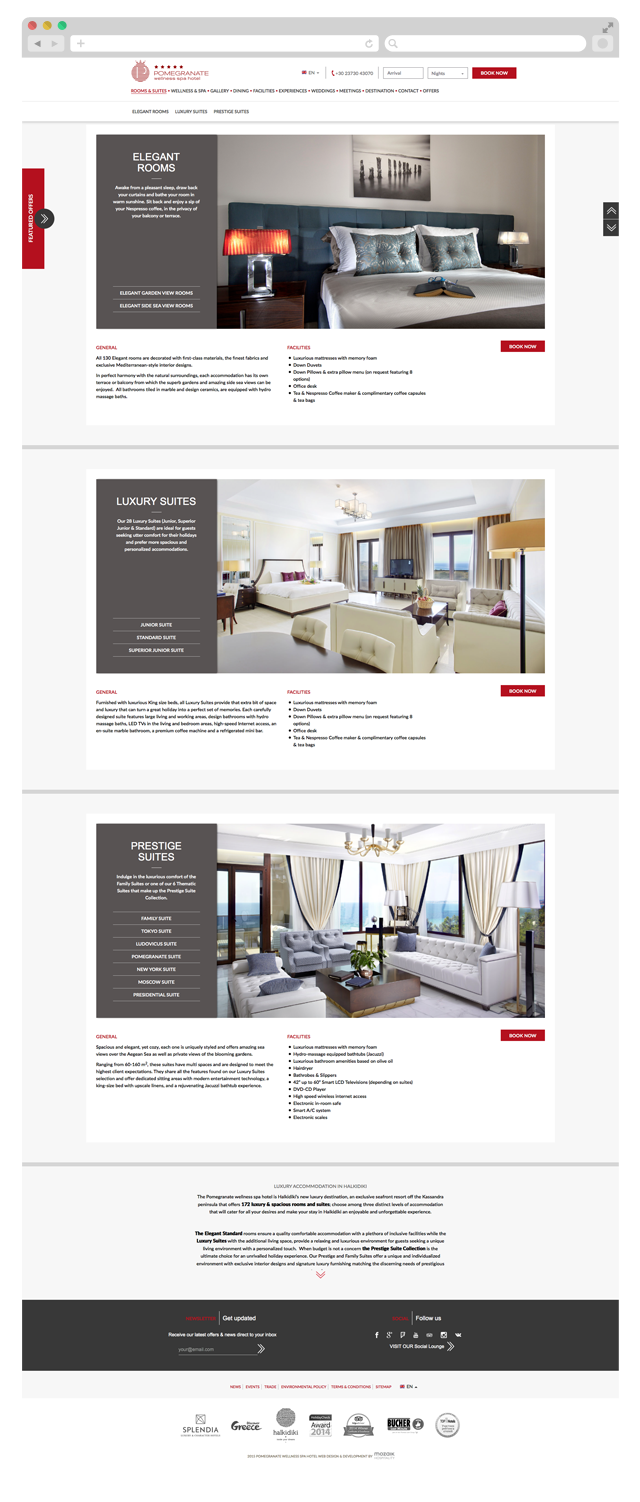This image showcases the homepage of a website named "Pomegranate." The site features a circular red logo with a white "P" at its center. The page is dedicated to "Elegant Rooms" and displays a well-decorated bedroom. The room includes two side lamps on nightstands, a mattress adorned with a white cover and four pillows, a book paired with a set of blue glasses, and a blue headboard. A piece of art hangs on the white wall, adding to the room's aesthetic.

Further down the page, details about the facilities are listed, along with options for "Luxury Suites," which depict a larger, more spacious room furnished with a couch and a wooden table. There is also information on "Prestige Suites," featuring a living space characterized by numerous windows and doors, providing an expansive and luxurious atmosphere.

The webpage predominantly features a clean white background. At the bottom, a dark bar houses various logos offering additional information about the company.